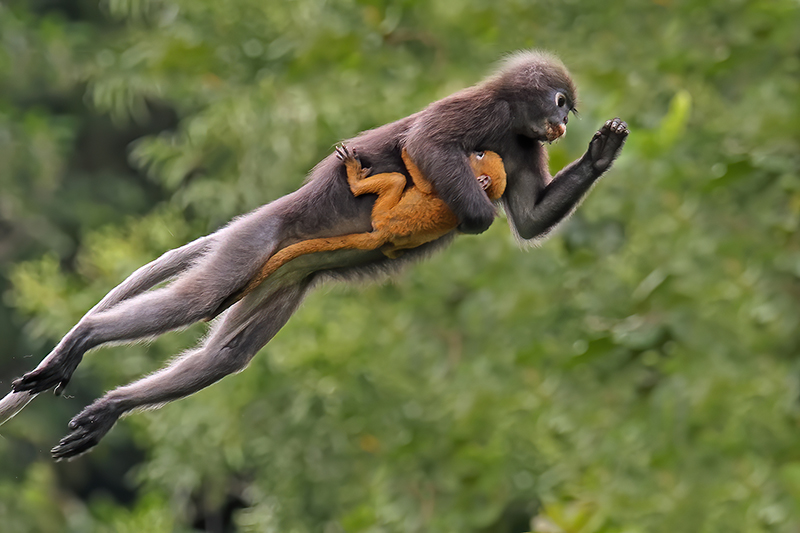The image features a dynamic scene of a mother monkey, grayish-brown with a long tail, leaping through the air to the right, while holding a smaller, bright orangeish-red baby monkey close to her chest with one arm. The mother's feet are positioned in the lower left of the image with her head in the upper right. Her left paw is outstretched in front of her, and her right arm securely supports the baby monkey. Both monkeys are in sharp focus, contrasting with the blurred background comprising a canopy of tree leaves in varying shades of green. The baby monkey, visible with its left eye, ear, leg, and foot complete with long talons, clings to the mother, intertwining its tail with hers. The background imagery suggests a lush, forested environment, further accentuating the sense of motion and maternal care depicted in the photograph.